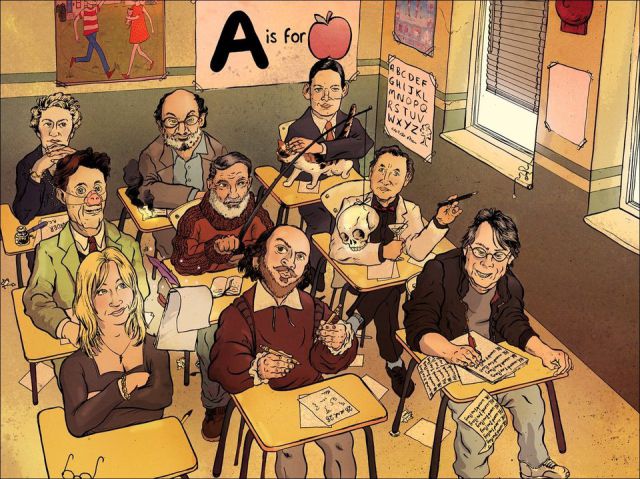This detailed watercolor illustration features a whimsical classroom scene filled with various renowned authors. The setting is a mock schoolroom, complete with old-fashioned single-seat desks with tabletops. In the forefront, a figure resembling Stephen King furiously scribbles on sheets of paper, discarding each page onto the floor in a frenzy of creativity. Beside him, a character that unmistakably resembles William Shakespeare gazes thoughtfully upwards, holding a pencil in each hand, perhaps contemplating his next great work.

To Shakespeare's left sits a blonde woman, who also appears to be an author, although her identity remains elusive. The classroom is filled with other famous writers, their faces faintly familiar, adding to the literary ambiance. This scene, rendered in soft watercolors with detailed pencil and pen work, captures the essence of literary genius and the studious atmosphere of a bygone educational era.